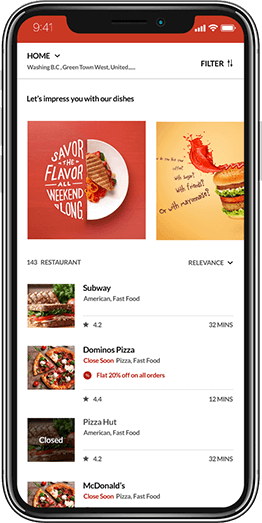The promotional image is designed to mimic the screen of a cell phone, complete with visible borders and bezels. The display features a restaurant location app, although the app's name is not shown. At the top, a red banner hosts the phone's notification status bar, with white text indicating cell data, Wi-Fi coverage, battery life, and the time, which is 9:41.

The main section of the app displays a white background with black text. The home location is set to Washington, D.C., or possibly B.C., with further navigation options like Green Town, West, and United States listed. The tagline "Let's impress you with our dishes" is prominently displayed above vibrant images of red and orange food items, enticing viewers.

Below these images, the app lists four fast food restaurants in the area: Subway, Domino's Pizza, Pizza Hut, and McDonald's. This organized layout suggests the app is tailored for users seeking quick dining options.